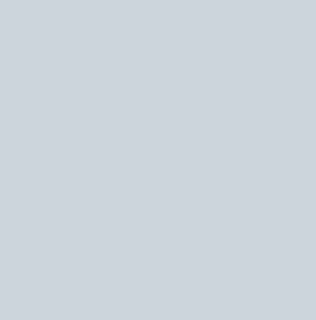The image depicts a small, uniform box centered on an otherwise white page. The box appears to be a blend between gray and a subtle mint green, creating an ambiguous hue. There are no visible elements within the box, such as text or titles. The color fills the entire box uniformly, suggesting it might be a minimalistic digital artwork or a simple graphical element.